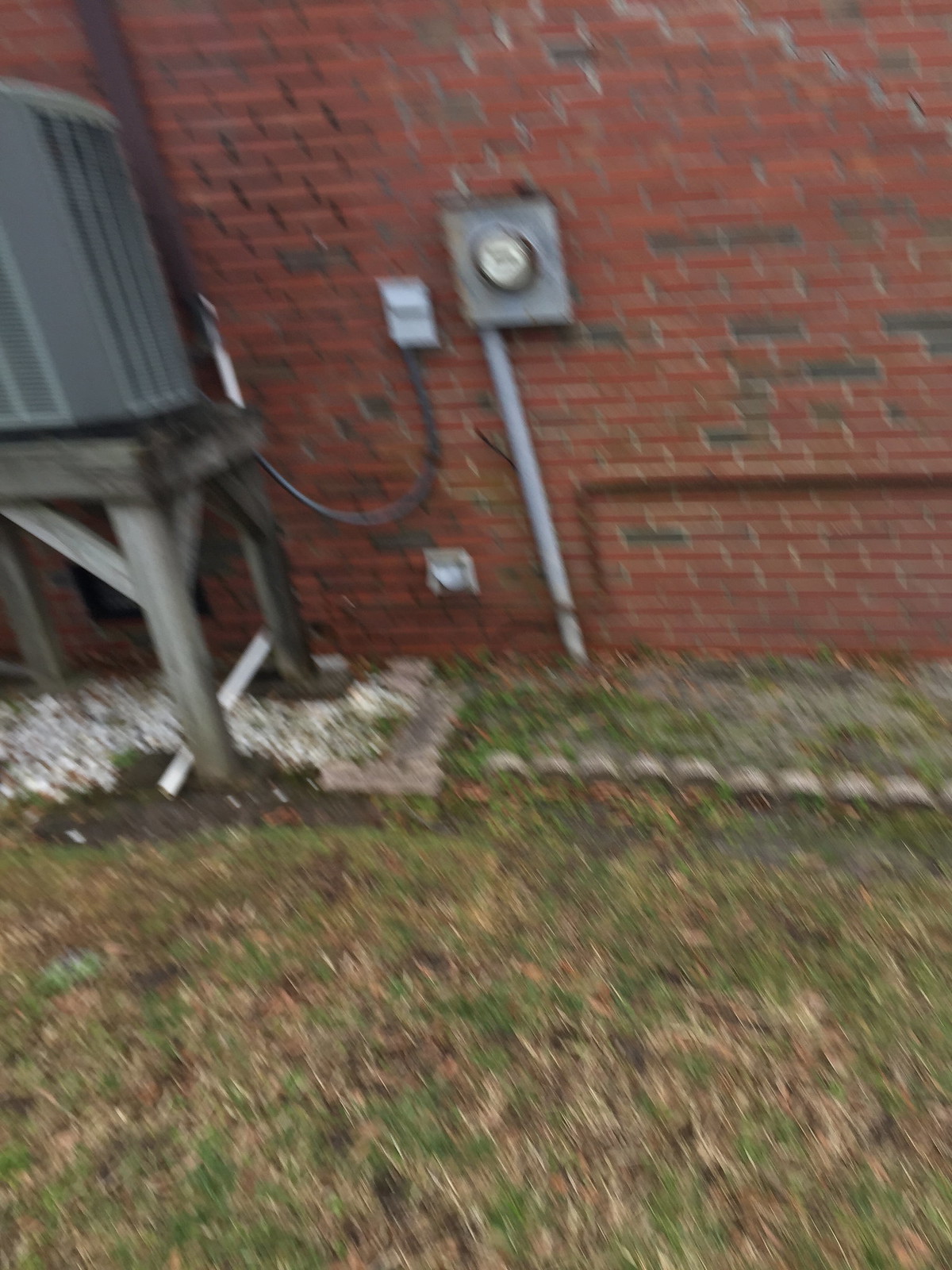A bright, clear day illuminates a red brick wall adorned with a gray power meter prominently attached to its surface. Extending down from the meter is a metallic pole reaching all the way to the ground. To the left, a gray air conditioning unit rests on a sturdy wooden platform positioned just below the wall. The platform is flanked by neat patches of green grass and a bed of white rocks that sit directly beneath it. The red brick wall itself is tastefully interspersed with gray bricks, adding a touch of visual texture to the scene.